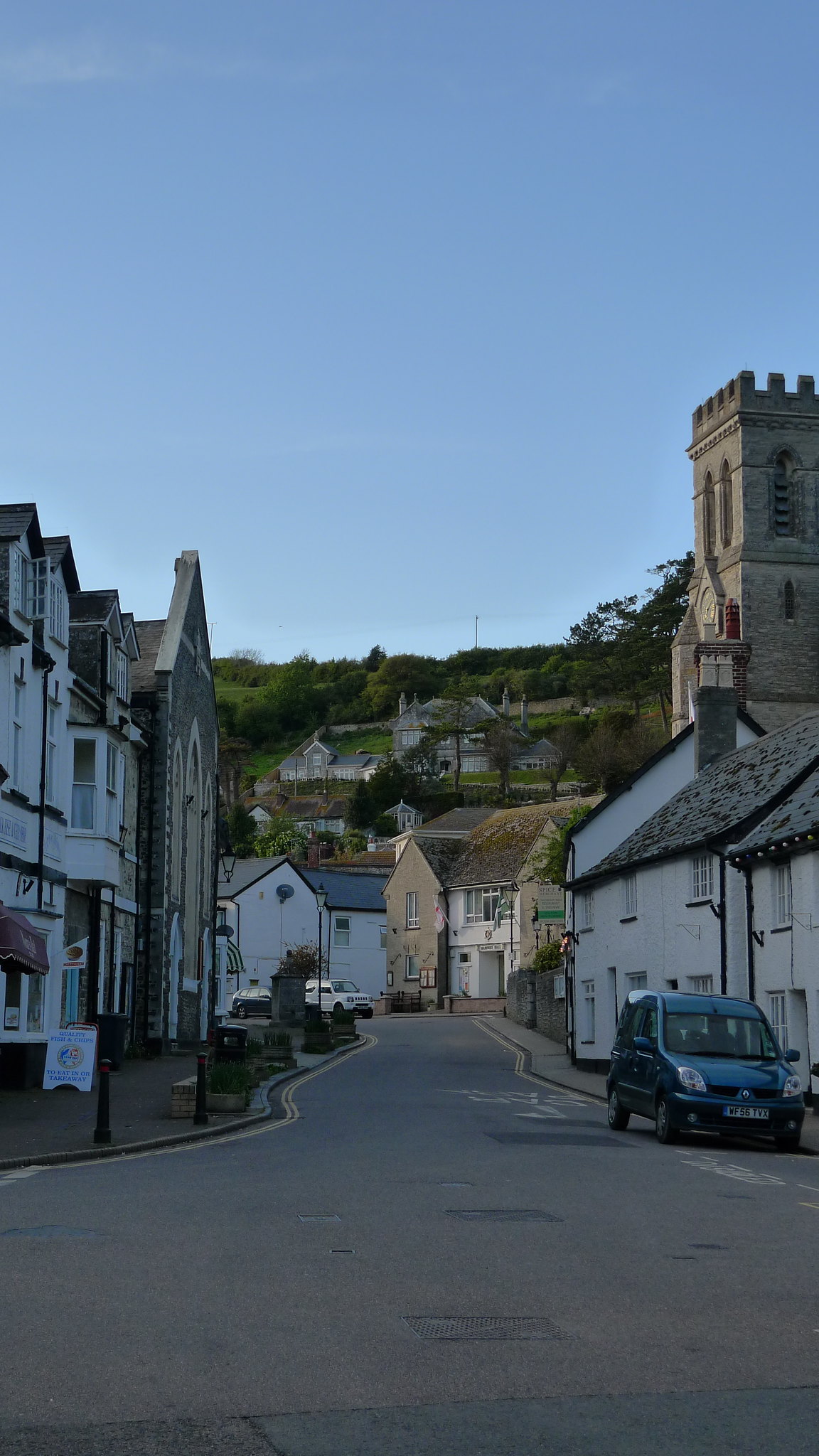The image showcases a charming European street scene in portrait view, with the top half dominated by a clear, beautiful blue sky. The bottom portion features a gray asphalt road that narrows into a smaller, ascending street flanked by old-fashioned, white, and brown buildings, some with arches and triangular roofs adorned with shingles. On the left and right sides of the road, there are sidewalks, a few cars, including a notable blue vehicle parked on the right side, and several posts and plants set in concrete areas. The road inclines towards a hill in the background, where more houses and a large castle-like building sit. The hill is dotted with greenery and trees, adding a natural touch to the architectural setting. The overall scene creates a picturesque blend of urban and natural elements, emphasized by the expansive, cloudless blue sky above.